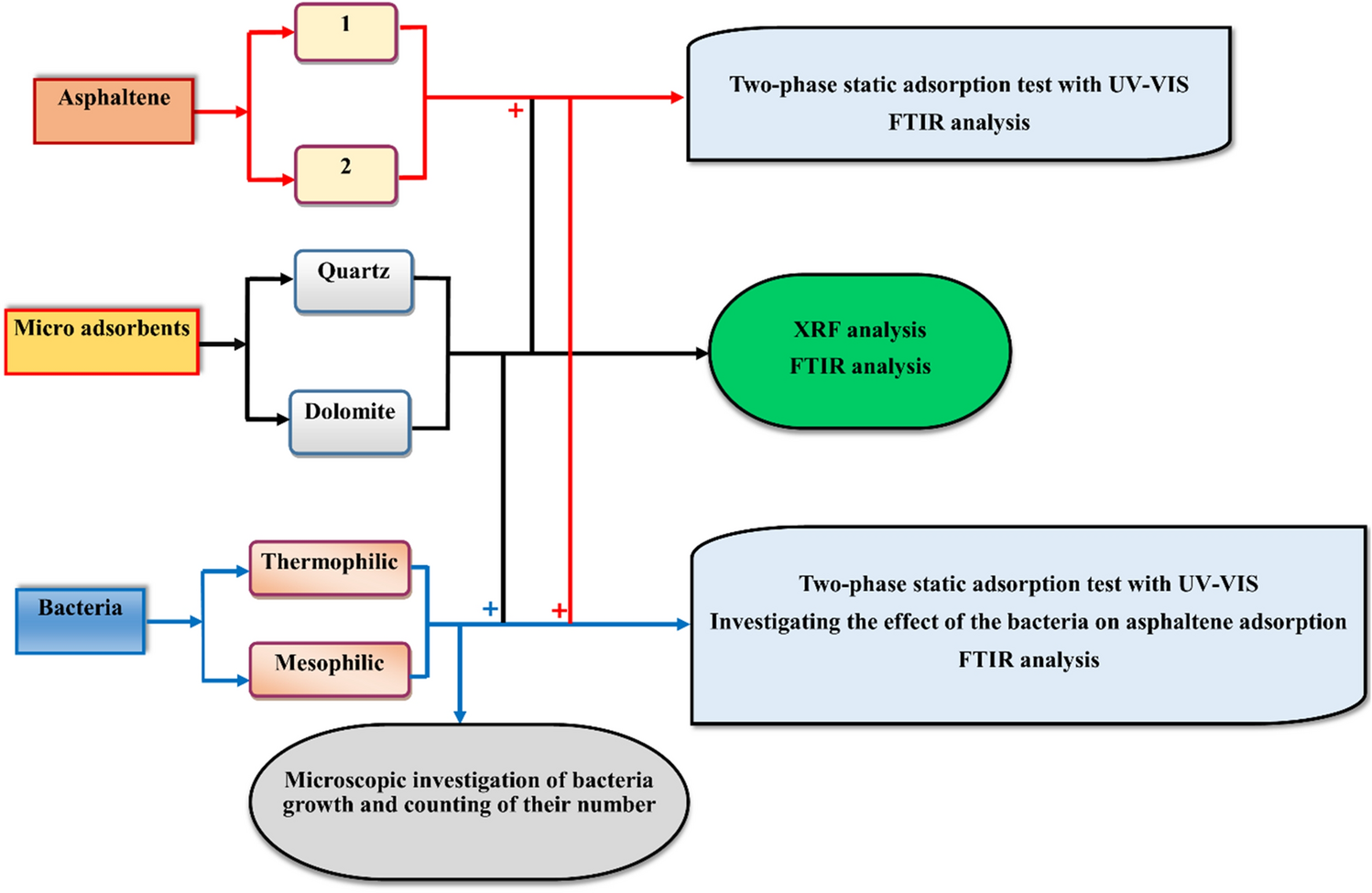This image displays a detailed colored flowchart diagram against a white background, illustrating various stages and components of a scientific analysis. 

On the left side, there are three primary headings within distinct colored boxes: an orange box labeled "ASPHALTENE," a yellow box outlined in red labeled "Microabsorbance," and a blue box labeled "Bacteria." 

The "ASPHALTENE" box has a red arrow leading to two green boxes labeled "1" and "2." The "Microabsorbance" section features a black arrow pointing towards two yellow-outlined boxes labeled "quartz" and "dolomite." Below this, the "Bacteria" box has blue arrows pointing to two black, pinkish boxes labeled "thermophilic" and "mesophilic," with a gray circle beneath stating "microscopic investigation of bacteria growth and counting of their number."

On the right side, arrows from these sections converge towards additional analytical steps. These include a gray box labeled "Two-phase static absorption test with UV-VIS FTIR analysis," a green circle indicating "XRF analysis," and a blue-gray box reiterating the "Two-phase static absorption test with UV-VIS investigation of the effect of bacteria on asphaltene absorption FTIR analysis."

This comprehensive diagram encapsulates the process flow from asphaltene separation and microabsorbance through to the microscopic analysis and various stages of UV-VIS FTIR and XRF analyses.